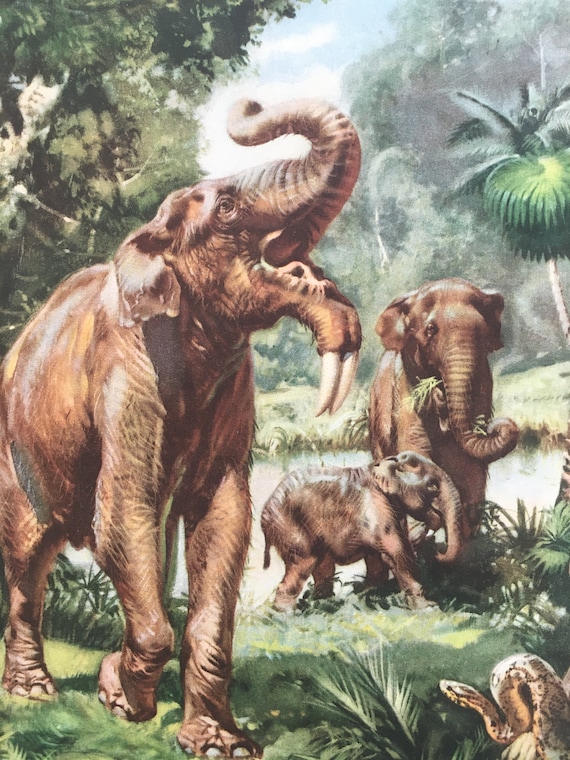The image depicts a rich, detailed painting of a jungle scene featuring three elephant-like creatures. The central focus is a large, brown, slightly hairy elephant with its trunk raised and mouth open, seemingly in distress or alarm. Uniquely, this elephant has tusks protruding from its chin, an uncommon feature for traditional elephants. The background showcases another adult elephant accompanying a smaller, juvenile elephant, both walking towards the right. The adult in the background holds grass in its trunk, suggesting it might be feeding. The lush setting includes verdant trees, shrubs, palm fronds, and a glimpse of a watering hole, evoking a jungle or savannah environment. On the grass-covered ground, a coiled snake poised near the bottom right appears to be the source of the larger elephant's agitation, creating a tense interaction in this vividly illustrated scene.